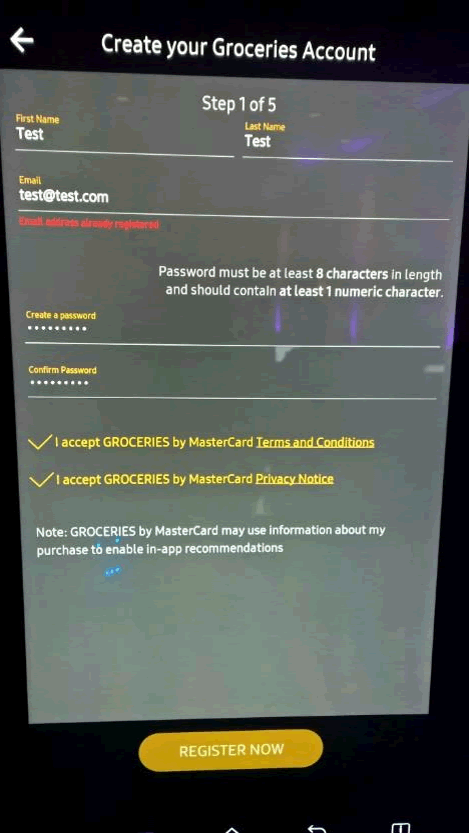This is a photo of a phone screen displaying a user interface for creating a "Groceries by MasterCard" account. At the top, there's a black bar with white text that says "Create Your Groceries Account." Beneath it, a gray, page-shaped rectangle spans the screen with the heading "Step 1 of 5."

This section contains several input fields. The first fields for "First Name" and "Last Name" are filled with "Test" in each. Below, there's an "Email" field with the placeholder text "test@test.com," followed by some unreadable red text due to the poor image quality. Further down, there's a note stating, "Password must be at least 8 characters in length and should contain at least one numeric character."

Below this note are fields for creating and confirming a password. Further down, in yellow text, it says, "I accept Groceries by MasterCard Terms and Conditions." Another line underneath states, "I accept Groceries by MasterCard Privacy Notice." Finally, at the bottom in white text, it reads, "Groceries by MasterCard may use information about my purchases to enable in-app recommendations."